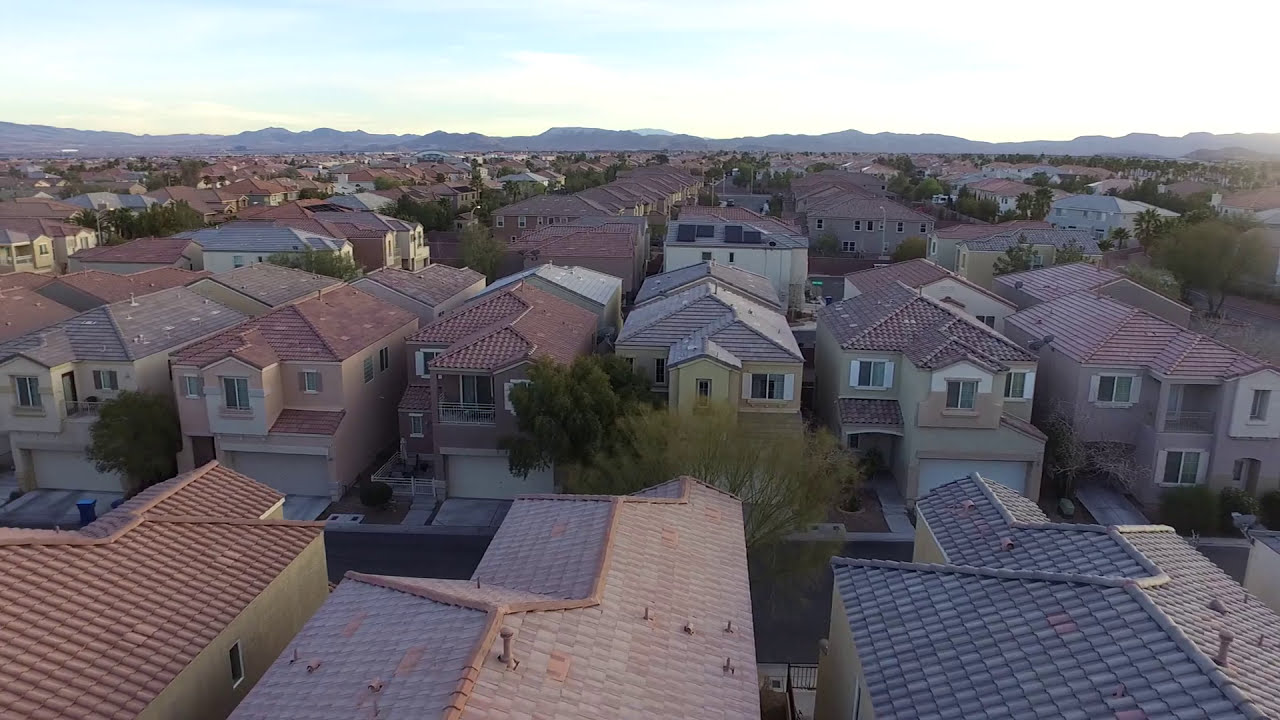This image captures a densely packed neighborhood of newly constructed, two-story single-family homes lined up along a street. Each house features similar architecture but varies in roof color, showcasing an array of pink, blue, and red tile roofs, with one house having a distinctive black roof. The homes also differ in exterior paint, ranging from beige to peach to gray. Each home has three front-facing windows and a small deck over the garage.

The street runs horizontally across the lower portion of the image, flanked by rows of these houses that continue in a repeating pattern far into the distance. There are a few trees scattered along the first row of houses, with more trees placed sporadically in the background. The closely situated houses, with only a few feet between them, stretch back almost to the top of the image.

Beyond the rows of houses, a flat expanse of land appears, framed by a mountain range in the background. The mountains, though not very tall, create a picturesque backdrop against the blue sky, dotted with white clouds. The setting suggests a hot, arid climate akin to Las Vegas or Arizona. The streets in the neighborhood seem devoid of cars, save for a few scattered trash cans, reinforcing the impression of a newly finished subdivision awaiting its first inhabitants.